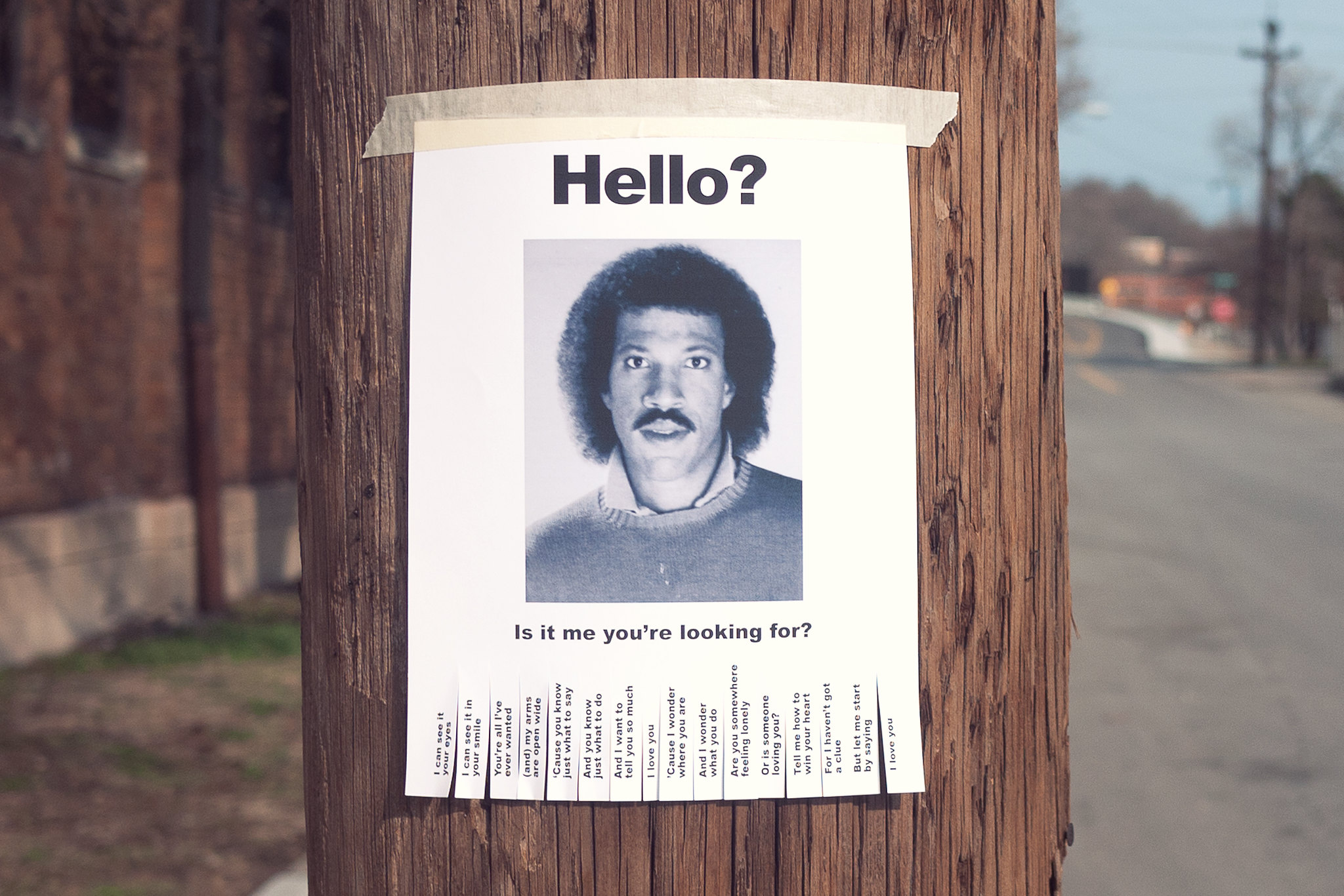This image depicts a humorous, nostalgic scene combining elements of pop culture and everyday life. Central to the image is a photograph of the iconic singer Lionel Richie, famous for his soulful ballad "Hello." In the photograph, Richie is sporting an afro and a mustache, dressed in a collared shirt layered with a sweater. The picture is taped to a wooden telephone pole using masking tape, reminiscent of old-fashioned “missing” or “for sale” signs. Surrounding Lionel Richie's image are the bold letters "HELLO?" At the bottom, it reads, "Is it me you're looking for?"—a lyric from his famous song. The setup evokes a sense of nostalgia and humor, paralleling traditional tear-off signs, but instead of phone numbers, passersby are meant to tear off strips of paper containing lyrics from the song. The background reveals a street, a patch of grass, and other indistinct urban elements, grounding this playful tribute in a everyday setting.